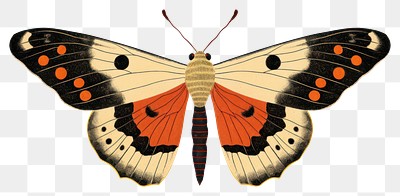This image is a type of clip art, depicting a butterfly against a grey and white checkered translucent background. The butterfly is centrally positioned, facing upwards with symmetrical wings resembling those of a monarch. Its body is striped, featuring a light brown top section with even lighter stripes and a black and red striped lower section. The butterfly has two long antennae and black circular eyes. The wings are divided into four sections: the upper wings are off-white near the body with black tips decorated with orange dots, and each has a single black circle closer to the body. The lower wings start with an orange section close to the body, bordered by black, transitioning to a beige or off-white color towards the tips, which are also edged in black with three distinct black dots each. The intricate lines on the wings highlight the different portions, and the image has an ink splatter effect, making it suitable for various advertising or web design projects.